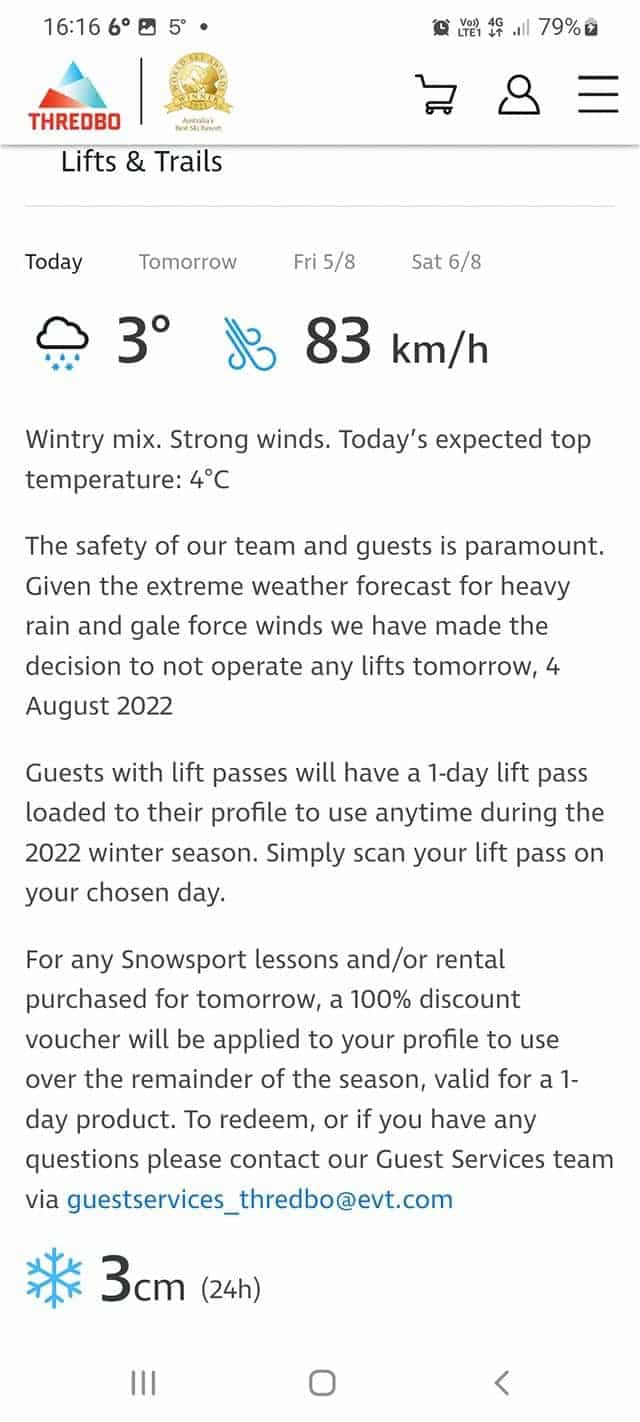Screen capture of a weather forecast on an iPhone, showcasing crucial weather-related information and operational updates. 

The upper part of the screen features the standard iPhone ribbon and navigation buttons at the bottom. The central area is dominated by today's weather forecast with three tabs at the top indicating different days: "Today," "Tomorrow," "Friday 5/8," and "Saturday 6/8," suggesting that the current date is in August.

The weather icon displays a rain cloud, indicating rain, accompanied by a temperature of 3 degrees Celsius. Adjacent to this is an icon representing wind with a noted speed of 83 kilometers per hour, signifying a particularly windy day.

The forecast further specifies harsh conditions: "Wintery mix, strong winds." Today's expected high is 4 degrees Celsius.

Below this, an important notice is provided:

"The safety of our team and guests is paramount given the extreme weather forecast for heavy rain and gale-force winds. We have decided to not operate any lifts tomorrow for August 2022. Guests with lift passes will have a one-day lift pass loaded to their profile to use anytime during the 2022 winter season. Simply scan your lift pass on your chosen day."

For guests with snow sport lessons or rental purchases, a "100% discount voucher" will be added to their profile for future use within the season. The notice concludes by advising guests to contact the guest service team for any inquiries.

This detailed description efficiently conveys the weather conditions and operational measures taken for guest safety.